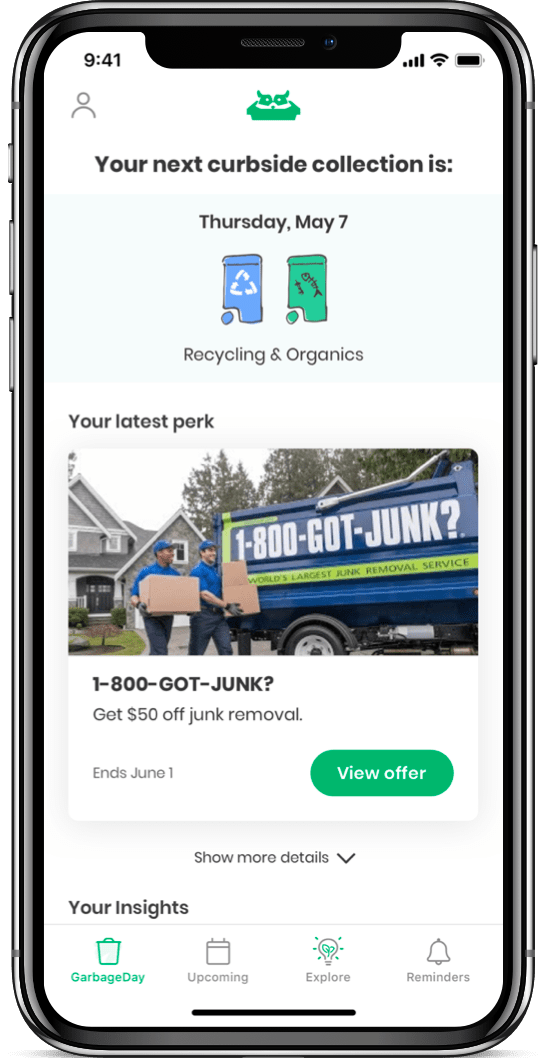The image shows a cell phone displaying an app interface on a white background. The screen provides detailed information about a user's curbside collection schedule from "1-800-GOT-JUNK." The app indicates that the next curbside collection for recycling and organics is scheduled for Thursday, May 7th. Additionally, there is an advertisement offering a 50% discount on junk removal services, valid until June 1st, with a green button labeled "View offer" in white text. Below the button, there is an option to "Show more details."

The app interface features a section labeled "Your Insights," with "Garbage Day" highlighted in green, while "Upcoming" and "Explore" are shaded in gray with green highlights. The bottom of the interface has a black line separating different sections. 

At the top of the screen, icons depict bins for recyclables and organics. The recycling bin is blue with a white recycling triangle symbol, and the organics bin is green, featuring a humorous depiction of a fish skeleton.